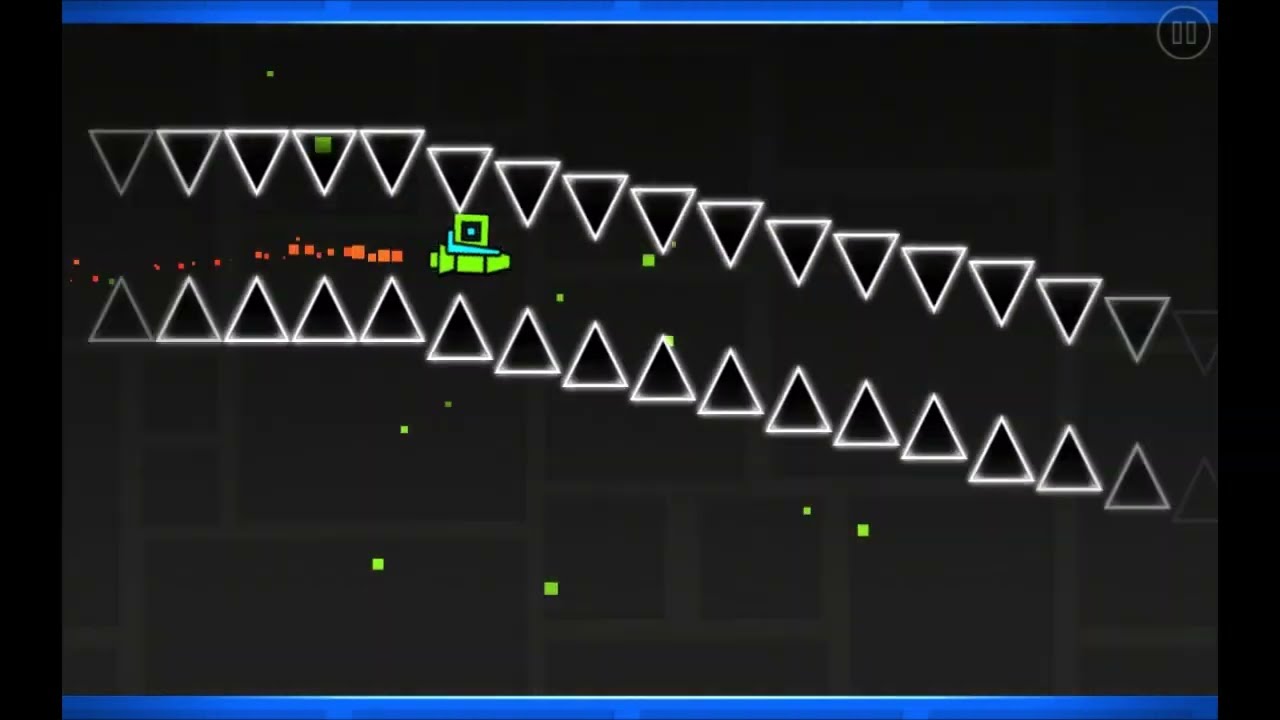The image depicts a horizontal rectangular screen, likely of a video game, featuring an animated green rocket ship flying through a geometric, dark gray and black cave-like background lined with connected square shapes of varying sizes. Framing the screen are blue horizontal bars at the top and bottom, along with thicker black bars on the left and right. The central focus is on two parallel rows of black triangles outlined in white; the top row of triangles is inverted, and the bottom row is right side up. These triangles converge slightly from the upper left towards the center right of the screen. In between the rows of triangles are a series of very small orange squares leading towards the green rocket ship. The rocket ship is detailed with a blue shape on its top and a green square marked with a black interior and a green dot at its center. Following the rocket is a red trail, and scattered around it are additional small green dots. Notably, a pause icon is visible in the upper right corner of the screen, hinting at the interactive nature of the scene.